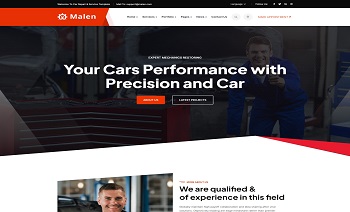**Descriptive Caption:**

The image is a screenshot of the homepage of a car repair and maintenance service website, showcasing a modern and professional design. At the very top, a red banner serves as the header, featuring the logo "Malin" on the left side. Navigation links to essential sections—Home, Services, Portfolio, Pages, Blog, and Contact—are also displayed, with icons for search, user account, and shopping cart positioned on the right.

The main focal area presents a large background image of a smiling mechanic working diligently on a car, set within a garage or workshop. Prominent overlay text in large white font reads, "Your car's performance with precision and care." Smaller text beneath this headline states, "Expert Mechanic Services." Two prominent buttons are available—an orange "About Us" button and a gray "Latest Projects" button.

The introduction section below features a split layout. On the left, there is an image of another smiling mechanic, while the right side contains text that begins, "We are qualified and of experience in this field." The rest of the text is cut off, but the design skillfully emphasizes the expertise and professionalism of the car maintenance services provided. Overall, the website layout is visually appealing, highlighting a commitment to quality and customer care in automotive services.